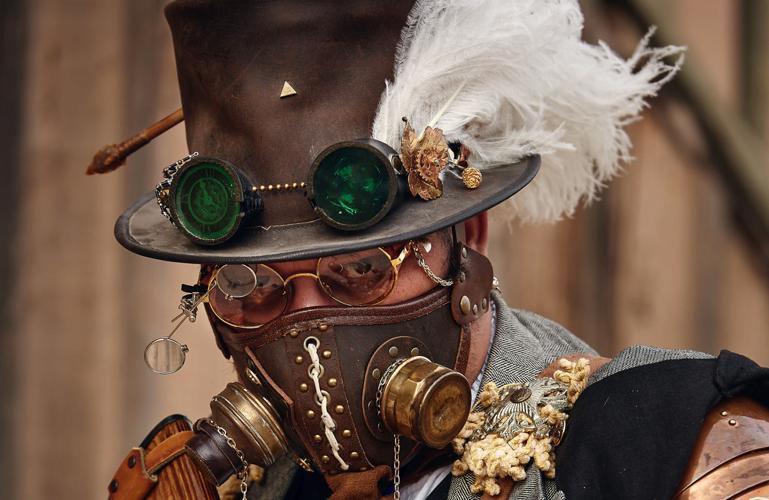The image is of a white man dressed in an elaborate costume, with the focus primarily on his head and shoulders. He is wearing a tall black leather top hat embellished with a white feather plume on the left side and an arrow sticking out from the right. Perched on the hat is a pair of dark green goggles. His face is adorned with round gold-rimmed glasses, with a smaller pair of bifocal glasses dangling from them. Covering his nose and mouth is a brown leather mask that resembles a breathing apparatus, equipped with two projecting prongs that look like metallic brass valves. He is also wearing a gray jacket with apparent labels on the shoulder and a piece of copper metal on the left shoulder. His attire is complemented by a demeanor of staring straight ahead, allowing a clear view of his eyes through the round glasses, but obscuring much of his facial features and the exact details of his body attire. The outfit hints at a mix of steampunk and possibly military influences, suggesting a character that might be part of a performance or a protest.